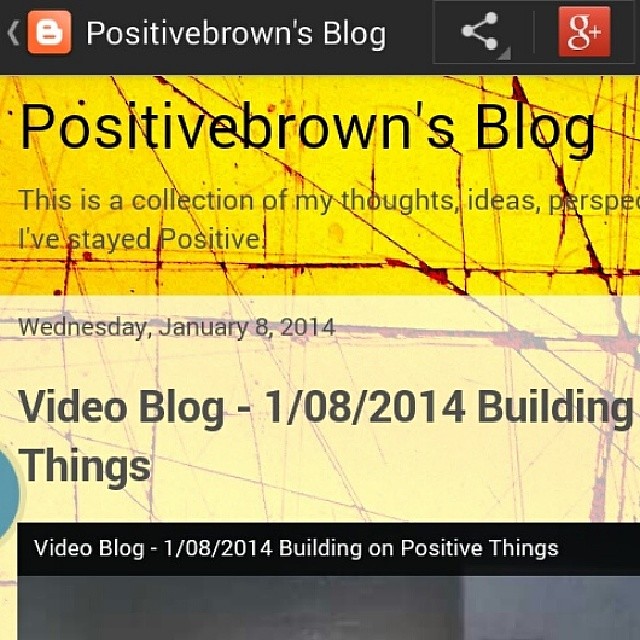The image is a screenshot of a website, specifically a blog hosted on Blogspot. In the top left corner, the Blogspot logo is visible, adjacent to the title "Positive Browns Blog." The top right corner features icons for sharing and Google Plus. The main header of the blog states "Positive Browns Blog" with accompanying text that reads, "This is a collection of my thoughts, ideas, perspectives. I've stayed positive." The date "Wednesday, January 8th, 2014" is also visible, followed by the title of a video blog post: "Video Blog 1-8-2014 Building Things." The background features a predominantly yellow hue with faint red lines, transitioning lighter towards the middle, and into a beige section towards the bottom. The top text is white set against a black background, contributing to a clean and crisp appearance.